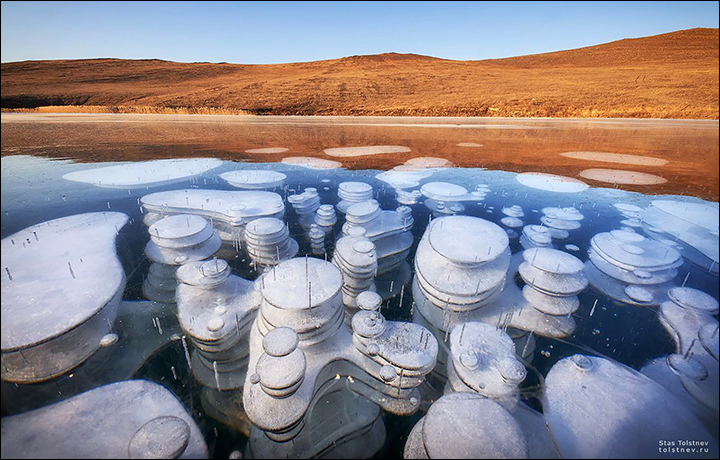This horizontally oriented photograph showcases a stunning outdoor scene of Lake Baikal in Russia. The crystal clear ice of the lake reveals mesmerizing bubbles of frozen methane beneath the surface. These bubbles, which appear as stacked whitish-blue disks, form intricate columns that descend deep into the water, resembling stacked shelves or concentric pads. The shapes of the bubbles vary, including round, oblong, and kidney-shaped forms. The clarity of the ice allows for an unobstructed view of these captivating formations. In the background, the landscape features gently sloping brown grassy hills leading up to a distant clear blue sky. Additionally, on the lower right-hand side of the image, there's a watermark indicating the photographer, Stan Tolstnev, and the website tolstnev.ru.